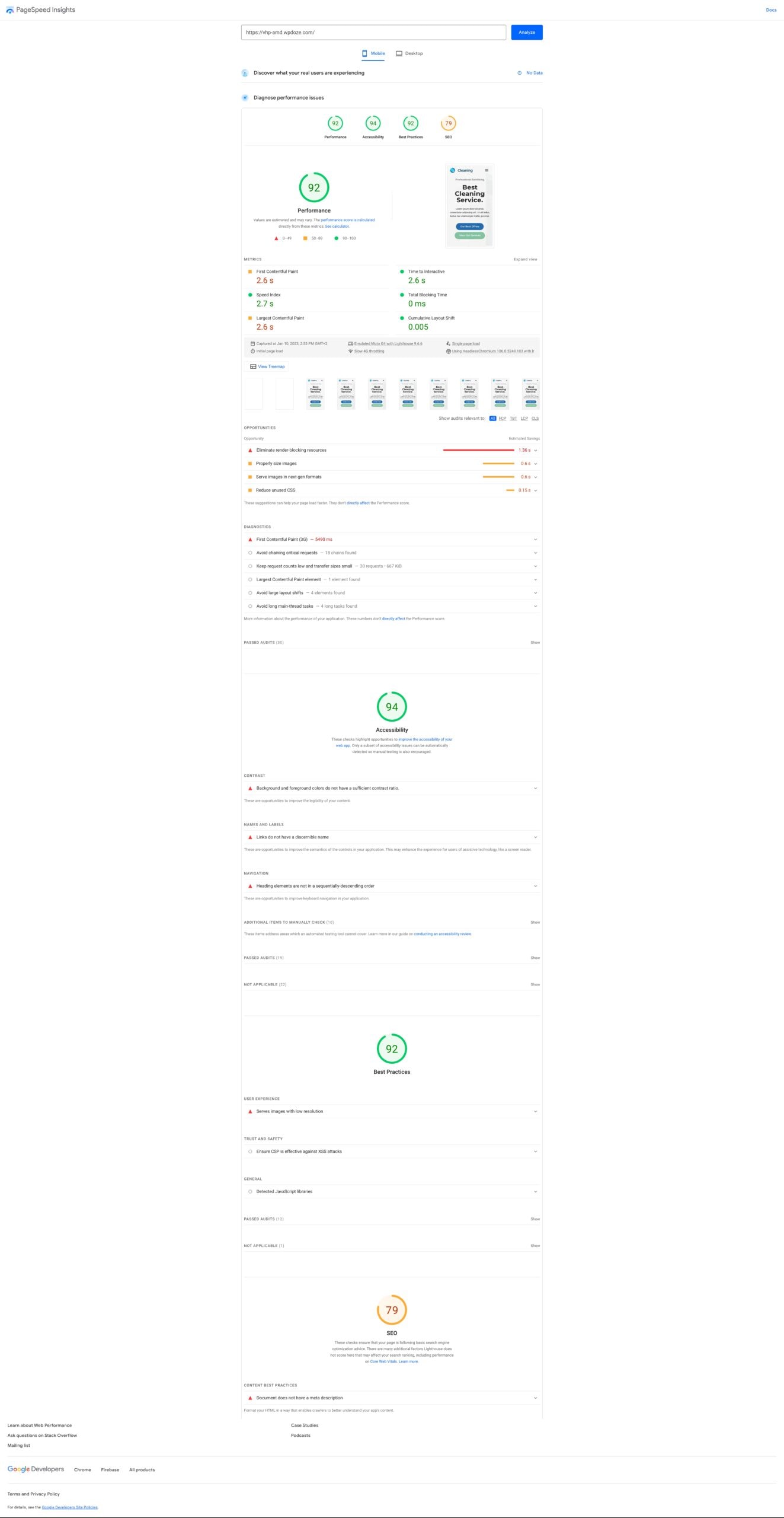This image depicts a vertical, rectangular document against a solid white background. The document appears to be a detailed data sheet or report and is fairly lengthy. At the very top, there is a search bar containing illegibly small black text, accompanied by a blue rectangular button featuring white text, though the exact words are unclear due to the image resolution.

Below the header, about an eighth of the way down, three small green circular icons followed by a yellow one are visible, each seemingly containing a number. As the eye moves further down the document, a larger green rectangular box appears, also containing a number, but again, the text is too small to discern.

Throughout the document, there is a lot of intricate data and detailed information, featuring predominantly black text interspersed with sections of green text for emphasis. Periodically, the document displays green circular icons with green rims, each containing a number with accompanying text beneath them. This pattern repeats itself multiple times down the length of the page.

Near the bottom of the document, another yellow circular icon can be seen, consistent with the color scheme and formatting present throughout the item. Overall, the document is rich with data and detailed elements, punctuated by green and yellow icons containing numerical information.